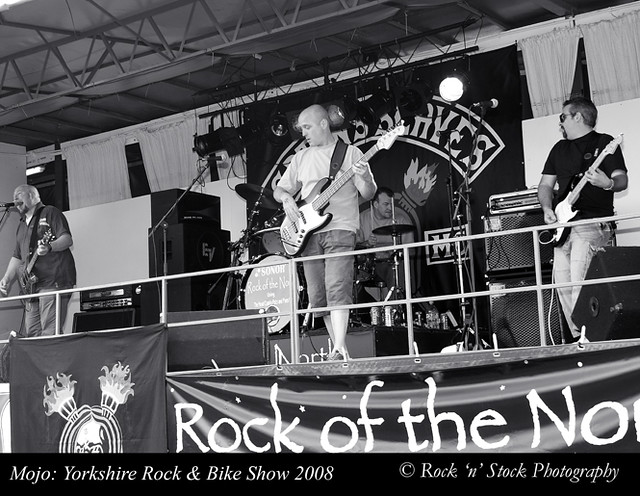This black-and-white photograph captures a dynamic live performance by a band on stage, likely taken during the Mojo Yorkshire Rock and Bike Show 2008, as noted by the text at the bottom of the image. The staged setup reveals ceiling bars and railings overhead, suggesting an indoor venue.

On the stage, there are four band members. To the far left stands a bald man in a polo shirt, who is playing an electric guitar and singing into a microphone. Centerstage, another man, who is partially bald and dressed in a short-sleeved shirt and shorts, also handles a guitar and sings into a microphone. Behind him, a drummer is visible, adding rhythm from his drum set. On the right side, a man sporting sunglasses, a black T-shirt, jeans, and a French beard, is strumming a guitar.

The backdrop features a stage curtain and an inconclusive banner, which likely reads "Rock of the North." Equipment such as speakers can be seen arranged around the stage, contributing to the concert ambiance.

The bottom of the image showcases a black horizontal strip containing the text: "Mojo Yorkshire Rock and Bike Show 2008" and "Rock and Stock Photography," providing context to this energetic snapshot of a live musical event.